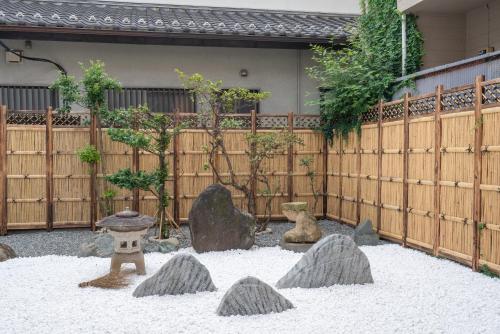The photograph showcases a meticulously maintained traditional Japanese Zen garden, surrounded by a tall bamboo fence. In the foreground, a white pebbly gravel area contrasts with larger, darker grey rocks, creating a serene landscape. At the center of this area, a small pagoda-like statue is nestled among the stones, evoking the calm ambiance of a temple. Toward the back of the garden, the gravel transitions to a greyish hue, and well-pruned, bonsai-shaped trees lend an air of tranquility. The garden is naturally lit, with the sunlight casting minimal shadows, suggesting a high sun position. The overall composition exudes peacefulness and order, characteristic of a well-kept Zen garden.